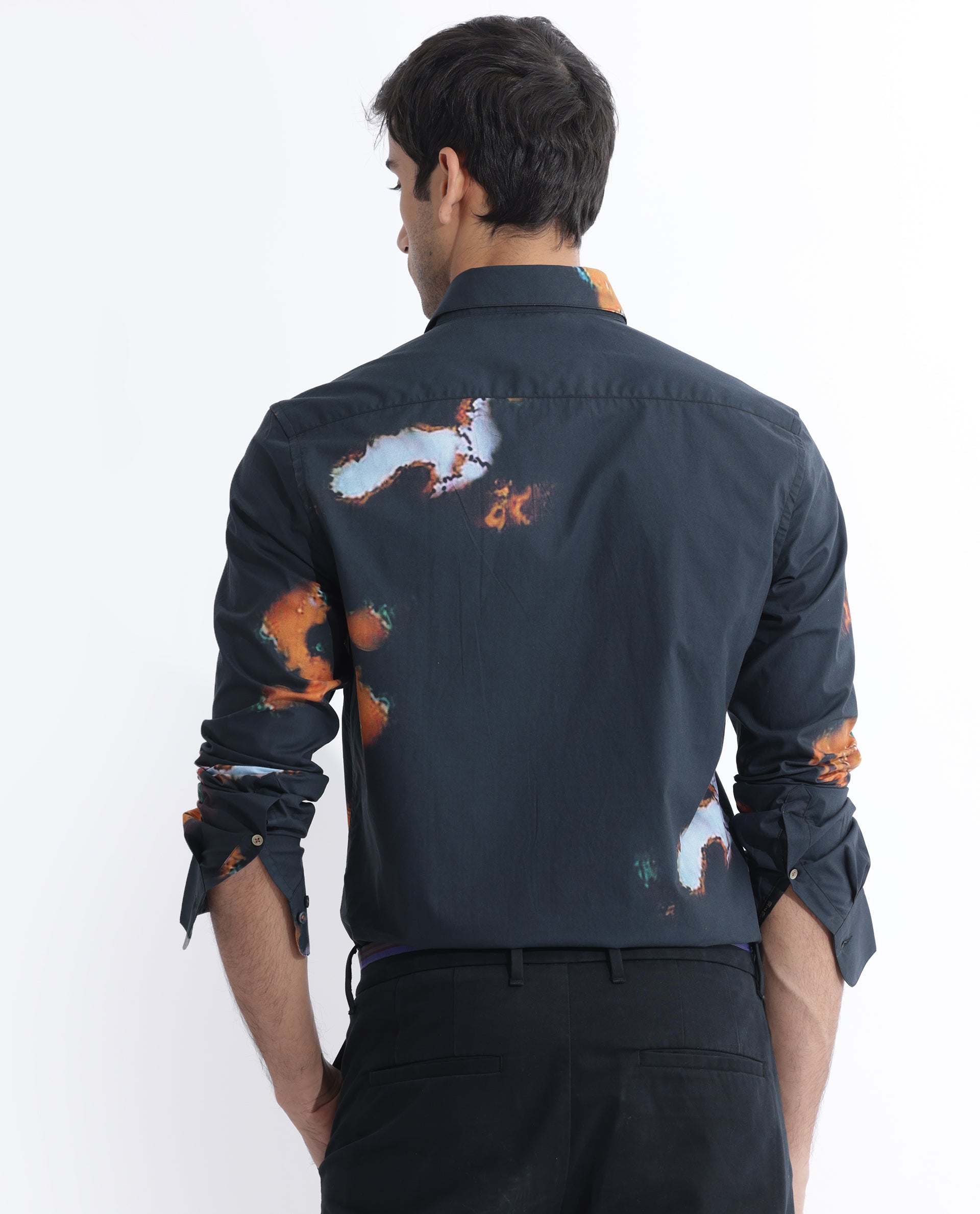This photograph features a young, light-skinned man with short, slightly messy, dark hair, standing with his back to the camera and his head turned slightly to the left. This positioning allows a glimpse of his nose, eyelashes, and the side of his face, revealing a bit of stubble. He is modeling a dark blue long-sleeved shirt that is characterized by several distinct splotches resembling bleach or paint stains. The stains are an eclectic mix of white, light blue, and orange, appearing on various parts of the shirt, including the upper left shoulder blade, the collar, the lower back, the sleeves, and the triceps area of the left arm. His sleeves are rolled up to his elbows, showcasing the veins on his right arm, and both sleeves are unbuttoned. His pants are dark, either black or dark blue, and one of his hands rests in his pocket while the other hangs by his side. The background is a simple, clean white, which emphasizes the details of his attire.